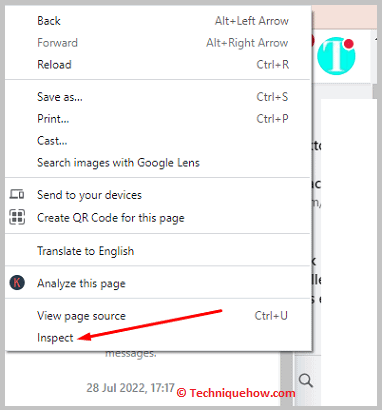The image showcases a screenshot of a website largely obscured by a pop-up overlay. The pop-up occupies most of the screen and offers several keyboard shortcuts and options for interacting with the webpage. The listed shortcuts and options are:

- **Back:** Alt + Left Arrow
- **Forward:** Alt + Right Arrow
- **Reload:** Ctrl + R
- **Save As:** Ctrl + S
- **Print:** Ctrl + P

There is also an option labeled "Cast," though it lacks a corresponding shortcut.

Following this, the pop-up introduces a section for "Search Images with Google Lens," succeeded by another section titled "Send to Your Devices." Below this, an option exists to "Create QR Code for This Page," illustrated with a square containing black squares.

Further options include:
- **Translate to English**
- **Analyze This Page** (indicated by a black circle icon with a red "K" inside)
- **View Page Source**
- **Inspect** (highlighted with a long red arrow and labeled with the shortcut Ctrl + U)

Below the pop-up, a limited view of the actual website is visible in the bottom right corner. Here, notable elements include:
- A large "T" within a teal box featuring a red circle
- Some textual content
- A search bar near the top
- A timestamp reading "28th July 2022, 7:17"

At the lower right, the web address is partially visible, reading "at technique.com" in red text.

This detailed caption encapsulates both the contents of the pop-up and the visible portion of the underlying website, providing a comprehensive description of the image.